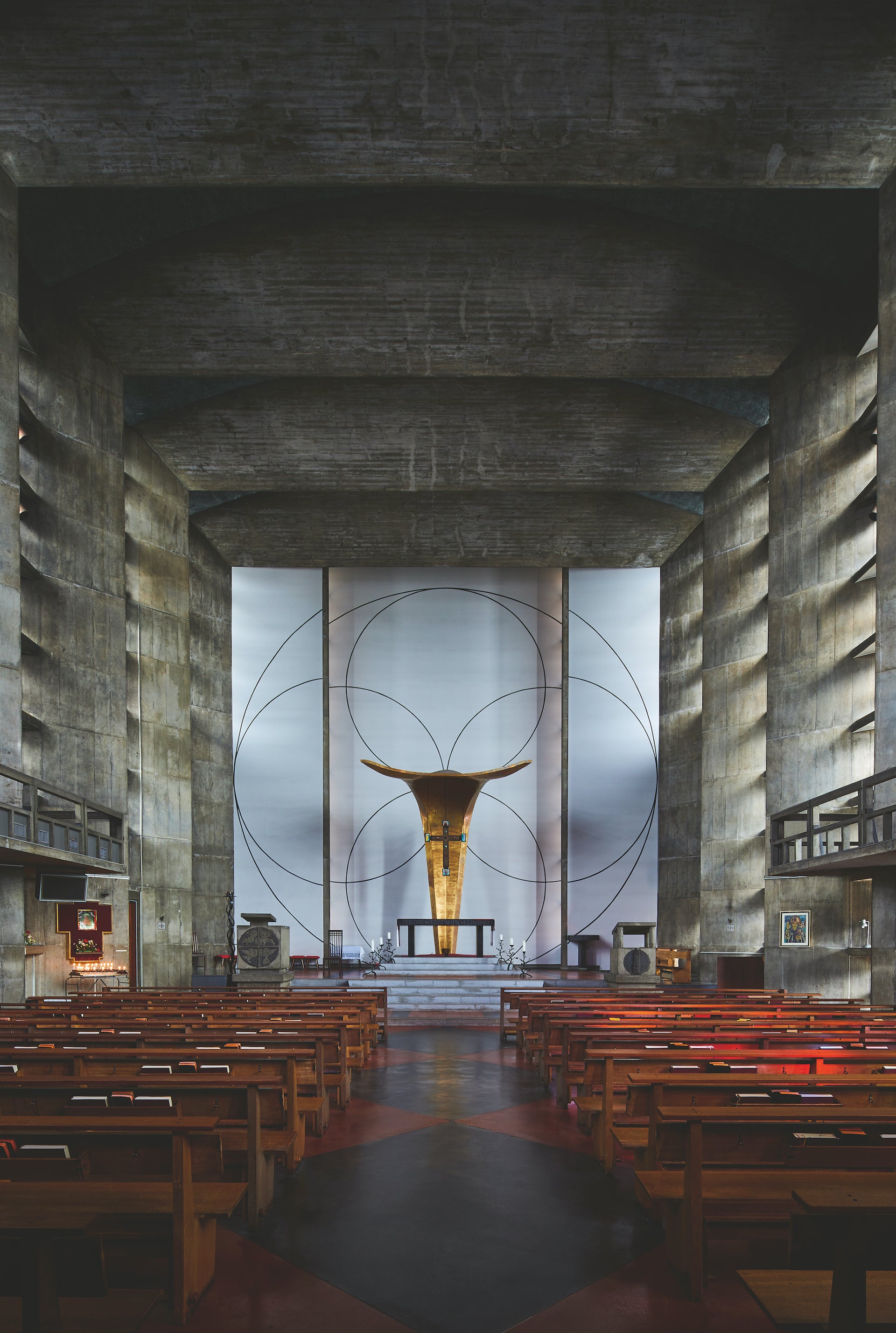The image captures the interior of an old, rustic church from the entrance, looking down the central aisle towards the altar at the back. The church exudes a dark and austere atmosphere with its tall, worn-out gray walls and dark-colored cement ceiling. The floor is also dark, in tones of red, complementing the overall somber palette. On either side of the aisle, rows of walnut-colored wooden pews line the space; nestled within their pockets are Bibles or hymnals, suggesting about 12 rows on each side.

The focal point at the end of the aisle is the altar, elevated by six or seven steps. Above the altar hangs a distinctive statue, which appears to be gold or yellow in color, tapering towards the bottom with arms extending horizontally, reminiscent of a human figure with outstretched arms. A dark-colored crucifix adorns this statue, framed against a blue background with a black outline design comprising concentric circles. The surrounding black outlines and quadrants add a stark contrast to the otherwise subdued tones. Alongside the altar, there are pulpits on both the left and right sides. The right wall features open shutters allowing in some light, breaking through the darkness of the concrete walls, lending a solemn yet serene atmosphere to the sacred space.